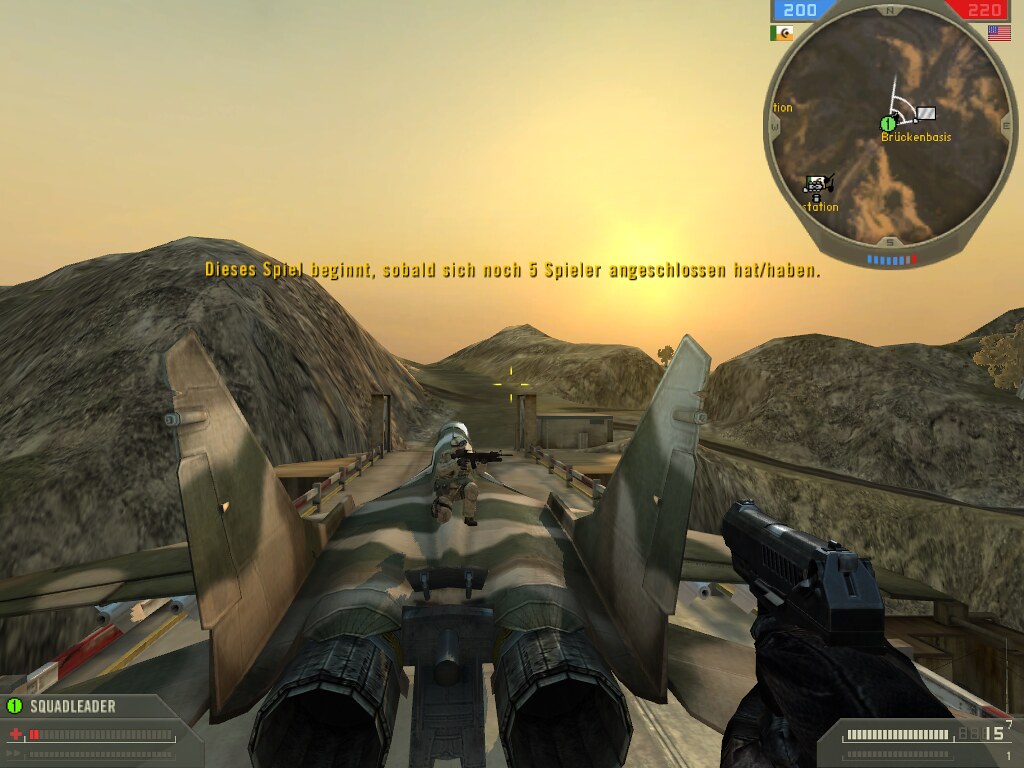This image captures a moment from a gameplay scene, full of in-game UI elements. In the bottom left corner, there is a label reading "Squad Leader" followed by the number "1". Directly below this, a prominent red plus sign is visible. Adjacent to the right, there are two red bars, further emphasizing their importance. Moving to the bottom right corner of the screen, a white bar is displayed with the number "15" aligned to its right. Centrally placed text reads "DIESES SPIEL BEGINNT, SOBALD SICH," suggesting a pivotal moment or instruction within the game. The image captures the anticipation and readiness associated with the start of the next gameplay sequence.